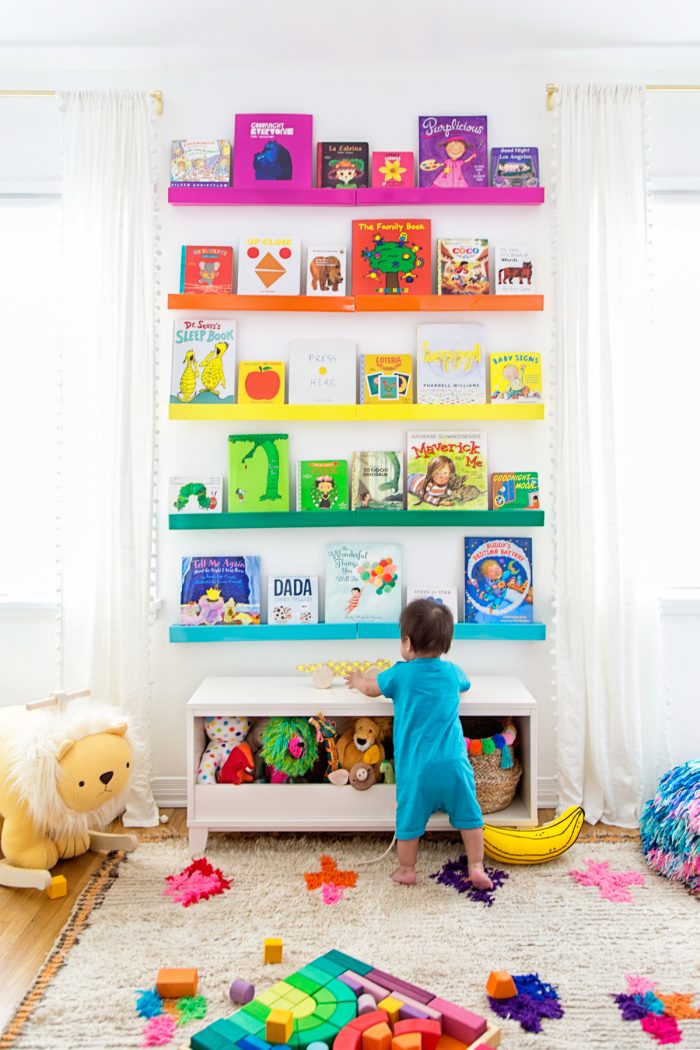The image depicts a colorful, brightly lit children's playroom featuring a small baby standing with his back to the viewer. The child, dressed in a teal onesie, is positioned in front of a toy shelf filled with stuffed animals, including a bear and two lions. Above the toy shelf are five bookshelves organized in a rainbow color scheme—magenta at the top, followed by orange, yellow, green, and blue—each adorned with books matching the shelf color. To the left of the baby, there is a fuzzy lion cradle, while the floor in front of him is scattered with toy blocks. The child stands on a carpet patterned with vibrant plus signs and near his feet lies a plush banana toy. The room also features two windows on the left, allowing natural light to brighten the space through white shades.